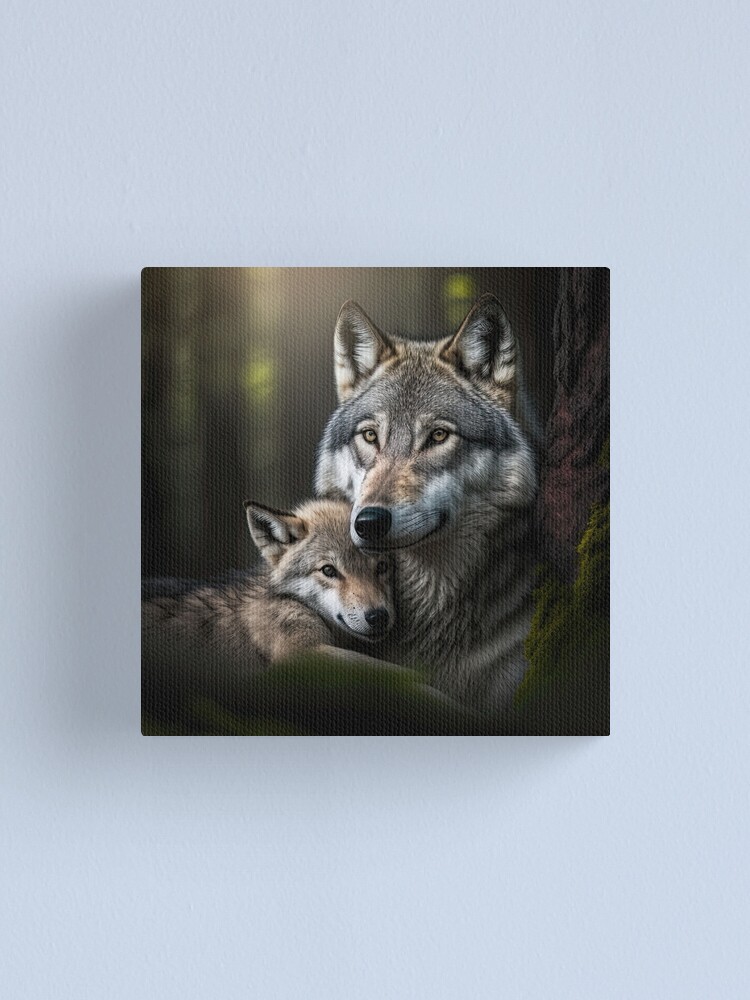This strikingly detailed photograph captures a deeply intimate moment between a mother wolf and her pup, set against a blurred, dark forest background with hints of green foliage. The image portrays a close-up of the mother wolf, positioned on the right and gazing into the distance, her fur a beautiful blend of gray, white, and subtle touches of brown around her nose and ears. The baby wolf, nestled closely against her, features more brown in its fur with patches of white on its face and snout. Their expressions and postures emanate warmth and tenderness, showcasing the loving bond between the two. The photograph is matted on a pale blue, almost sky-colored background, which frames the scene beautifully and makes the wolves stand out vividly. Additional details include the mother's green eyes, contrasting with the pup's brown, and a glimpse of a tree trunk in the upper right corner. The clarity and realism of the wolves, down to the fine details of their ears and noses, make this image both captivating and heartwarming.